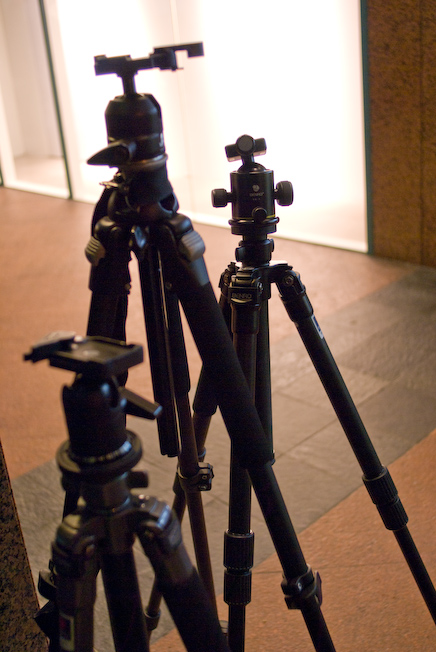In this detailed photo, three black ball head tripods are visibly standing on a red-brown tiled floor, each with three adjustable legs and empty mounts awaiting cameras. The floor alternates between the red-brown tiles and three rows of gray strips, adding contrast and cordoning off areas. The tripods are arranged in varying heights: the closest is the shortest, the middle one stands tallest, and the far one is intermediate in height. One tripod in the background features twist locks for leg adjustment, while the middle one utilizes clasp mechanisms. Behind the tripods, a modern interior can be seen with a mix of brown paneling and a glass partition or office wall that is slightly glazed, making it hard to see through due to bright light shining from the other side. There is also a marble wall to the left, adding to the contemporary setting. A beige-white wall with partially visible brown doors frames the background, completing the office environment’s aesthetic.